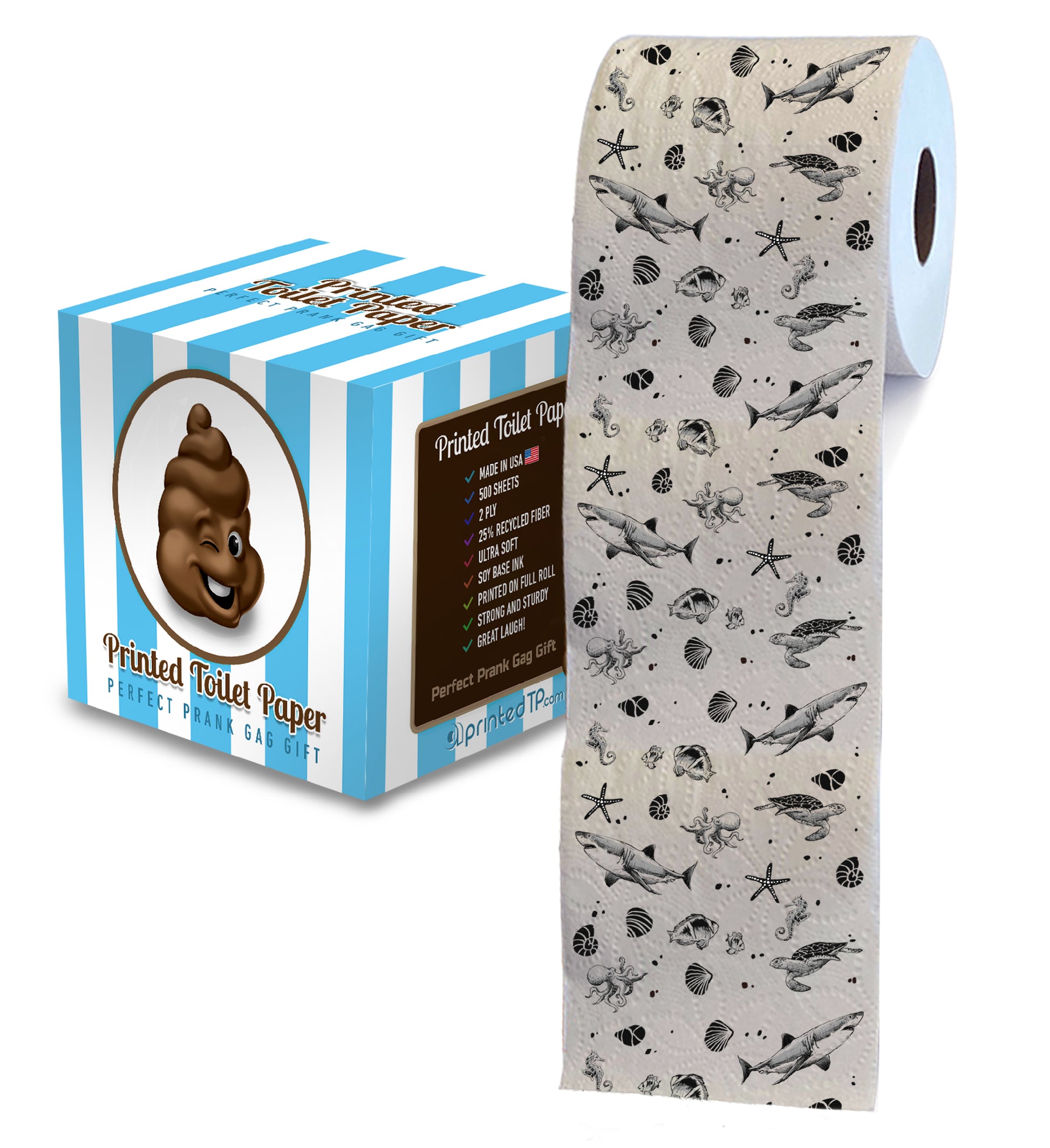The image showcases a roll of novelty toilet paper with an oceanic theme featuring black illustrations of sharks, starfish, regular fish, sea turtles, clams, seashells, and an octopus on white paper. The toilet paper exudes a "pretty" and "cute" whimsical charm, making it a perfect prank gag gift. To the left of the toilet paper, there is a blue and white striped box adorned with a cartoon poop emoji winking and smiling. Gold cursive letters on the box declare, "Printed Toilet Paper - Perfect Prank Gag Gift." Additional details on the box, including "Made in the USA," "500 sheets," "2-ply," and "25% recycled paper," emphasize the quality of this ultra-soft, humorous item.